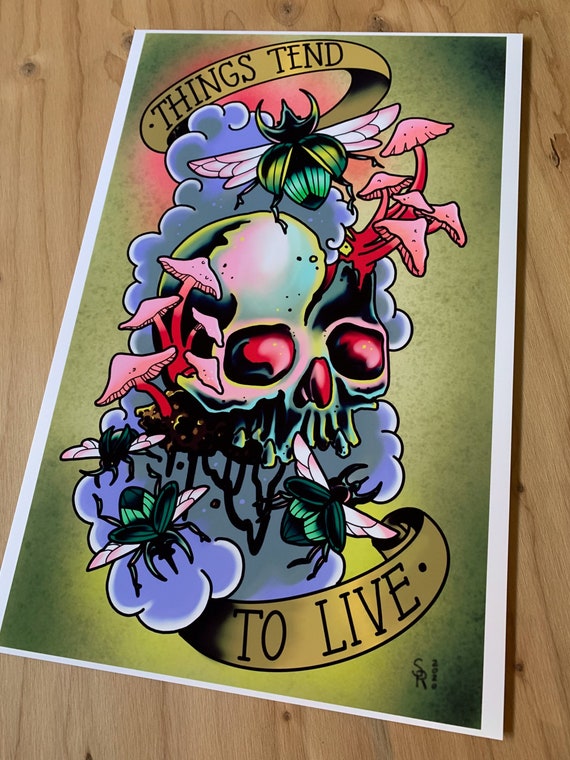The image depicts a computer-generated, traditional tattoo-styled illustration laid slightly askew on a light tan wooden table. At the top, a circular gold ring frames the text "Things Tend," while at the bottom, it reads "To Live." Central to the artwork is a skull with distinct red eyes and nose, adorned with vibrant pink and red mushrooms sprouting from the left side and right half. Perched on the skull is a green beetle with its wings spread wide, surrounded by additional beetles with dark green upper wings and light green underwings. The background features a swirling mix of blue-gray clouds and a sickly green, mottled with black, enhancing the eerie, vintage tattoo aesthetic. A small signature is visible in the bottom right corner of the print.